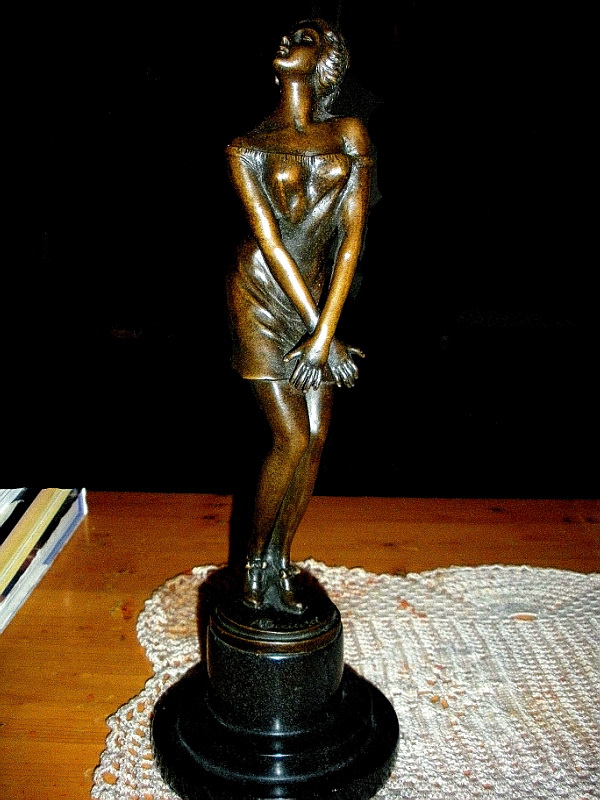The image features a detailed bronze-colored figurine of a woman, standing on a black base that appears to be made of either metal or hard plastic. The woman is depicted with short hair, arms folded in front of her, and is looking upward. She is dressed in a skirt with off-shoulder sleeves. The statue is situated on a wooden table, which is covered by a crocheted white doily. An etched inscription is visible near the feet of the statue, suggesting it might be an award. Adding to the scene, there are some books placed next to the statue. The background of the image is predominantly black, with lighting focusing on the statue and the table, indicating the photo was likely taken at night. The statue has hints of copper, bronze, and amber hues enhancing its metallic finish.